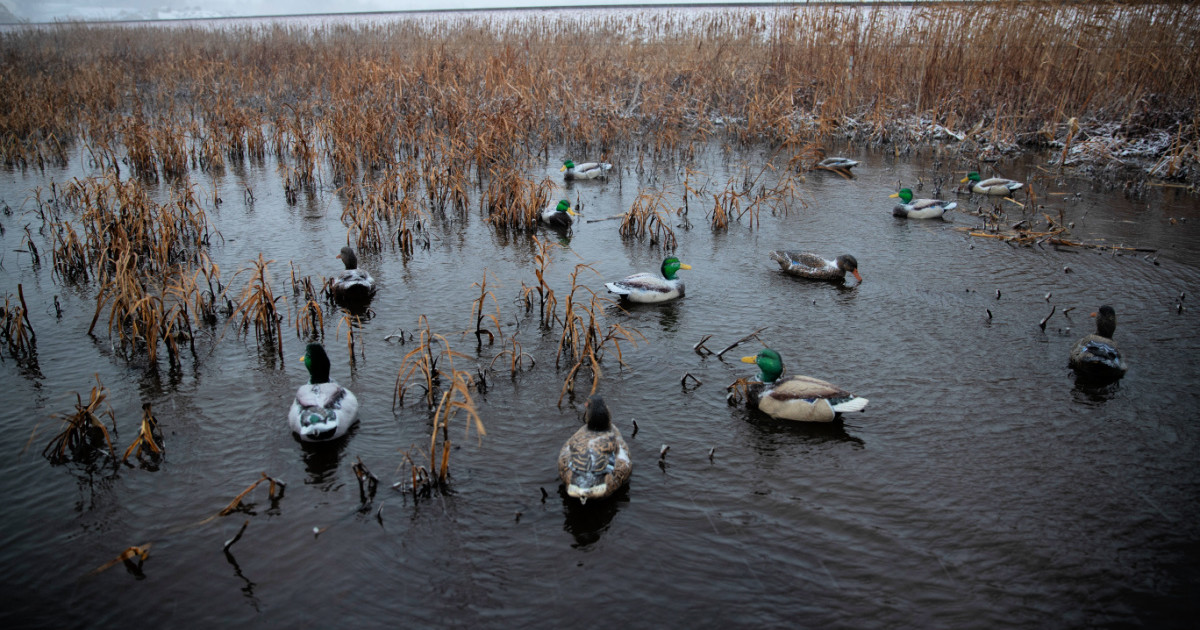This detailed photograph captures a serene, cloudy afternoon scene of a shallow pond surrounded by marshy land, dusted with a light layer of snow. In the water, a large group of approximately ten mallard ducks swim leisurely, their vibrant green heads and yellow bills standing out against their white, gray, and brown bodies. Some ducks exhibit a distinct dark brown stripe through their tan or gray feathers. The tranquil pond is dotted with tall, dead plants with light tan and gray hues, indicating a winter season. The ducks, scattered across the pond and seemingly relaxed, are either searching for food or possibly scouting for nesting spots in this picturesque natural habitat.